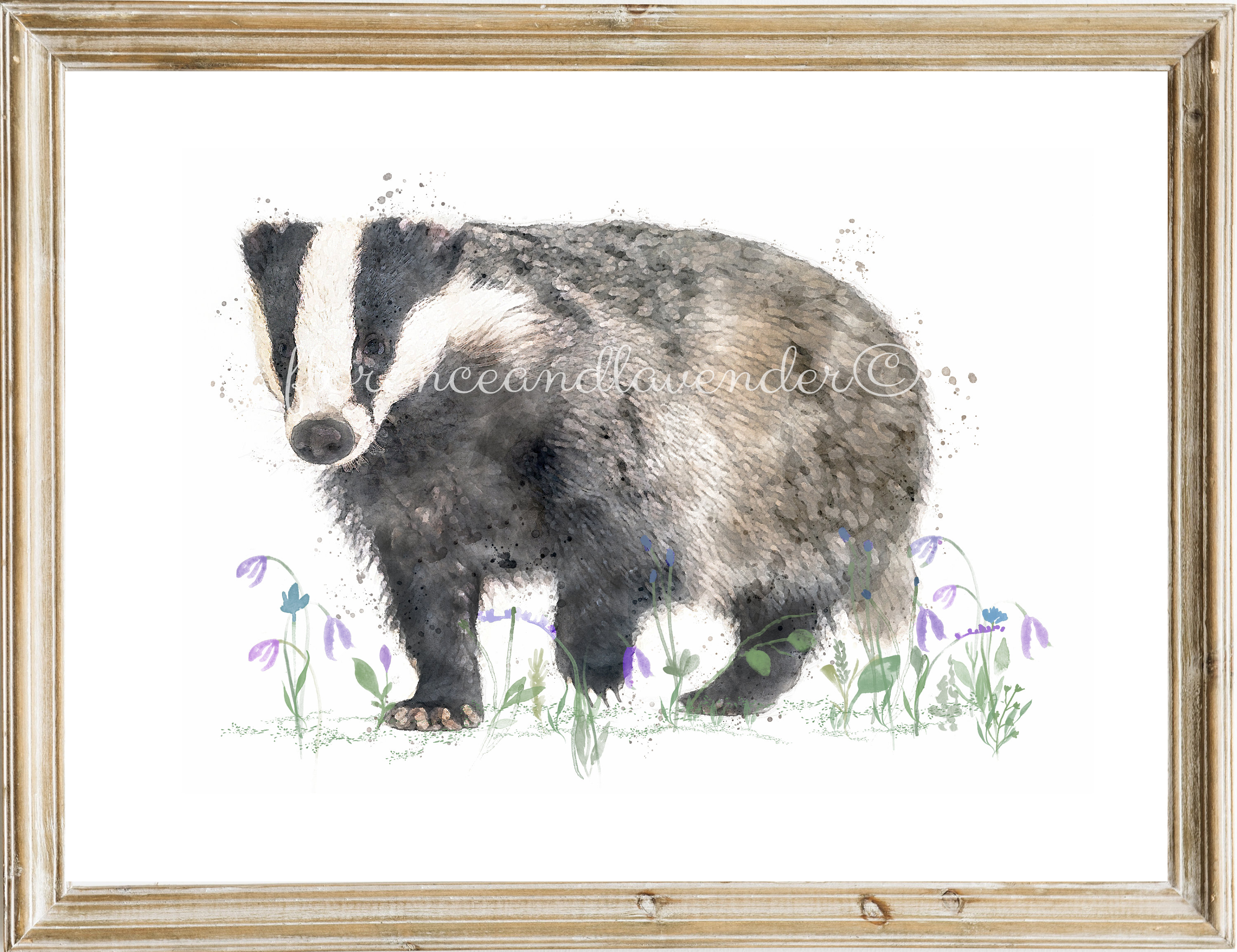This is a detailed framed painting of a badger, encased in a sleek, light brown wooden frame with visible knots. The painting features a badger on a white background, stepping amidst patches of green grasses and wilted purple and blue flowers. The badger has a distinctive appearance: its face is predominantly white with black stripes running over each eye, while its body showcases a mix of black with subtle transitions to dark brown and light white shades. The badger's stance is dynamic, with one front paw and one back paw raised, indicating motion. The artwork exhibits fine detailing with some speckled paint on the badger, suggesting a stylistic choice that mimics the texture of colored pencils or a digital brush. A barely legible watermark is present across the midsection of the badger, adding a layer of sophistication.